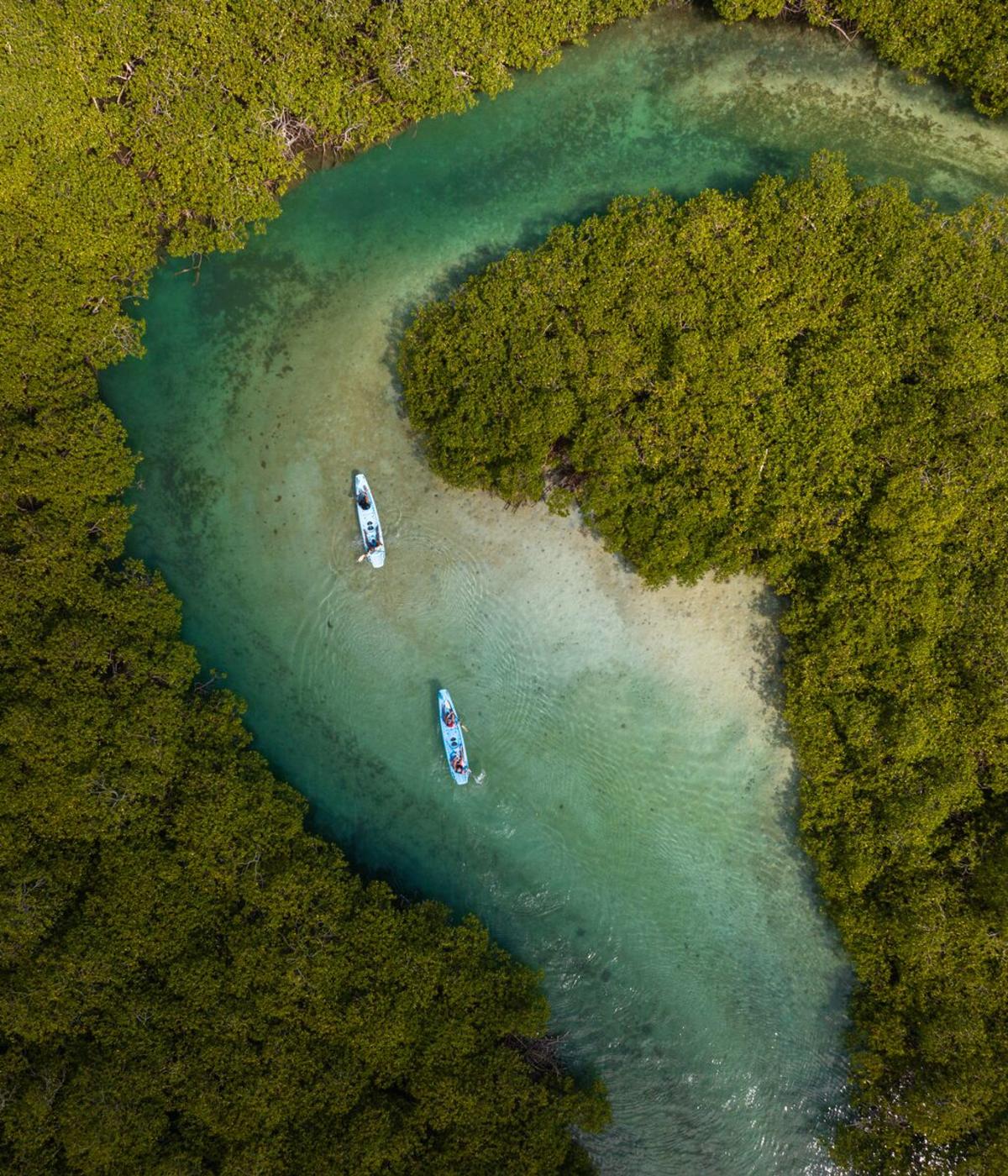This aerial photograph captures a winding river that starts in the top right corner of the image, curving down into a shallow, peaceful expanse of teal water with light beige marbling, and then narrowing again towards the bottom of the picture. The river follows a C-shape and is flanked by incredibly vibrant, dense green trees that create a lush frame around the water. In the river, two two-person kayaks, one light blue and the other appearing white, are visible. Both kayaks are elongated and thin, consistent with their design for smooth paddling. Each kayak has two occupants actively paddling with visible wooden paddles, leisurely navigating the calm waters. Beneath the surface, some mossy areas can be seen on the sandy riverbed, adding to the serene and picturesque nature of the scene.